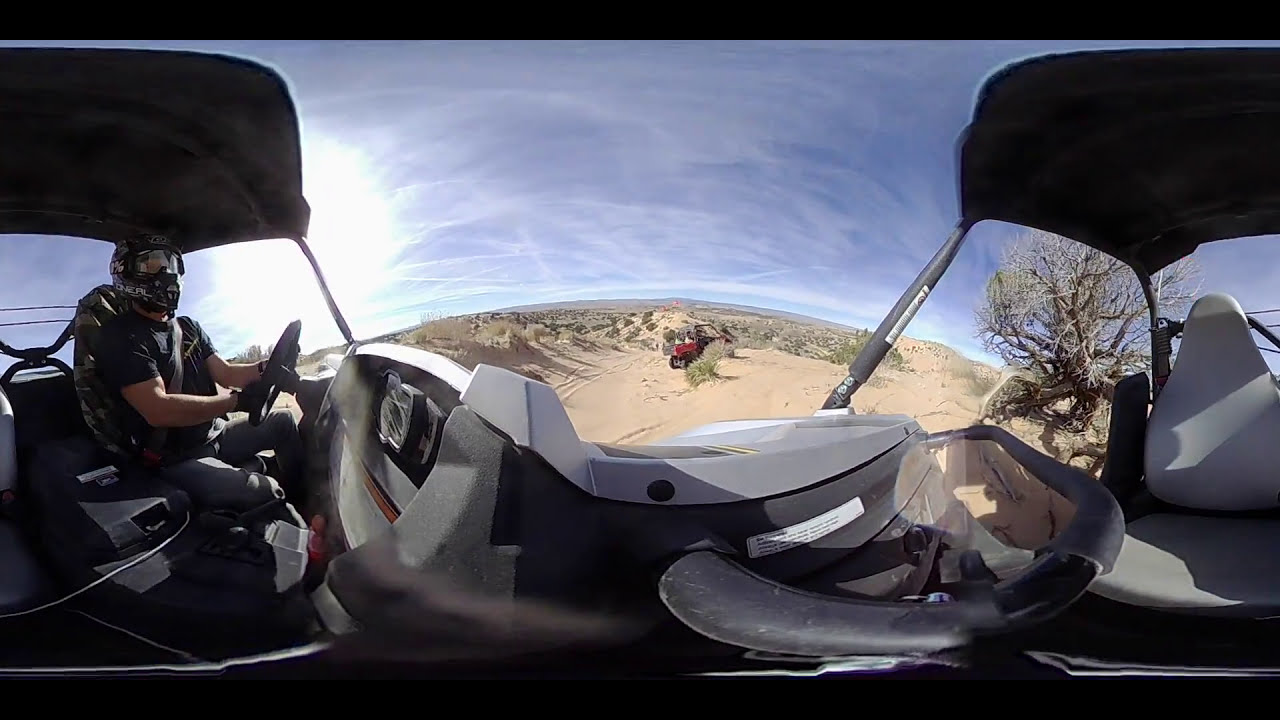In this outdoor scene, a man is driving an off-road ATV through a desert landscape comprising sand dunes and sporadic sagebrush. The driver, positioned on the far left of the image, is attired in a black helmet, black short-sleeve t-shirt, black gloves, and blue jeans. Seated with a seatbelt on, he grips a black steering wheel within the light and dark gray interior of the vehicle, which also features a black dashboard with various instruments. A protective metal awning covers the driver’s head, shielding him from debris and the sun.

To the right side of the image, another gray seat faces inwards, suggesting a multi-passenger capability. In the distant background, there's another ATV, this one red in color, as well as a third green four-wheeler.

The vast desert setting extends towards a distant mountain range under a sky that's light blue with streaks of cloudiness. Contrails from planes mark the sky, and the sun, partially hidden behind the light clouds, shines from the left side of the image.